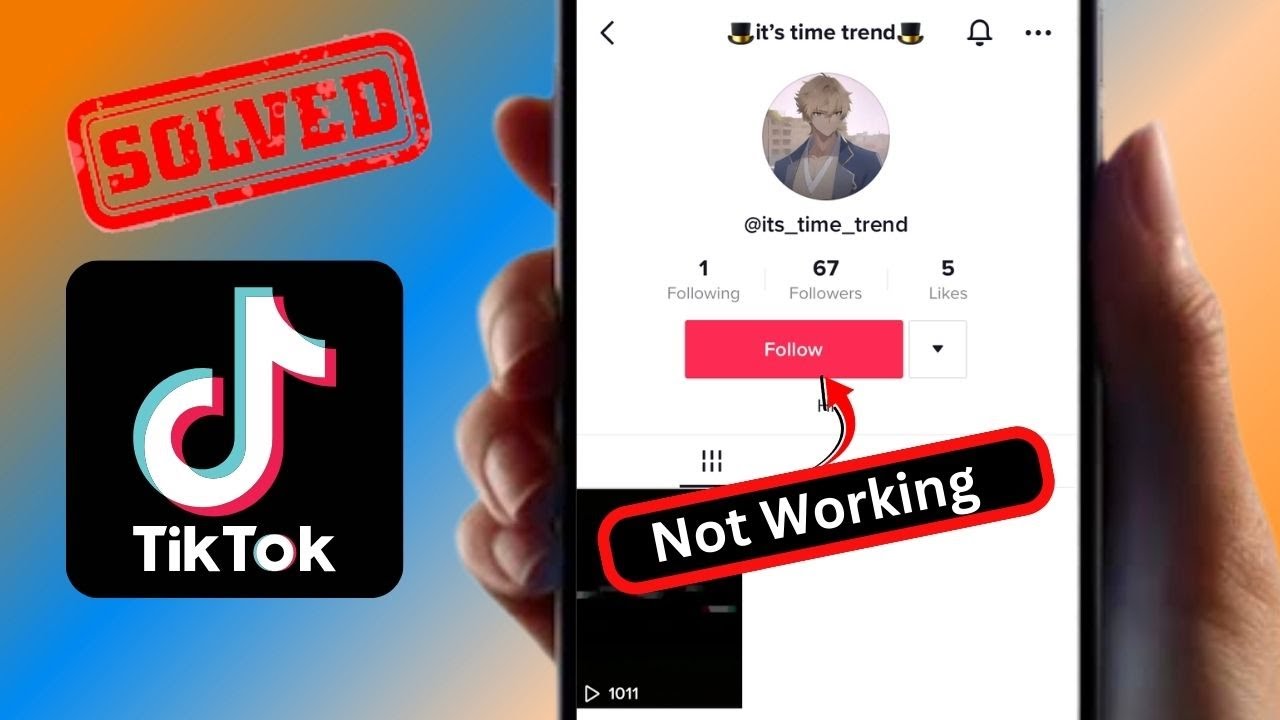This vibrant screenshot showcases a colorful graphic background with a rainbow gradient. The upper left corner features a red ink-stamp-style graphic with the text "SOLVED" in bold red font. Below this stamp, a black square prominently displays the Tic-Tac logo in white font.

To the right of these elements, a woman's hand is holding a smartphone with black bezels. The phone's screen has a white background. In the top left corner of the screen, there is a small black arrow pointing left. Centrally aligned at the top, two teacup emojis flank the text "It's time trend," which is followed by a bell icon and three horizontally arranged black dots.

Just below, a circle contains an image of a Final Fantasy Online character with gray hair. Directly under this image, the username is displayed in black font with the handle "@its_time_trend." Further details reveal the account is "following 1," has "67 followers," and has garnered "5 likes." Finally, at the bottom of the screen, a prominent red button with white font instructs users to "Follow."